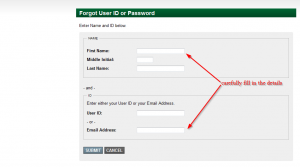The image features a user interface with a prominent, blurry visual and a green border at the top. The top section displays the text "Forgot User ID or Password" in a clear, bold font. Below this, on a white background, instructions are visible stating "Enter Name and ID Below."

In the middle of the image, there is a gray box, divided into two smaller sections. The top section is titled "Name" and further broken down into "First Name," "Middle Initial," and "Last Name," with corresponding text boxes to the right of each label. Below this, there is text that is not legible. Further down, instructions are provided to "Enter your User ID or your Email Address."

The next section specifies "User ID" with a text box for input, followed by "Email Address" with another text box beneath it. In the middle portion of the image, highlighted in red, there is an instruction stating "Carefully Fill in the Details," accompanied by red arrows directing attention to the "First Name" and "Email Address" fields.